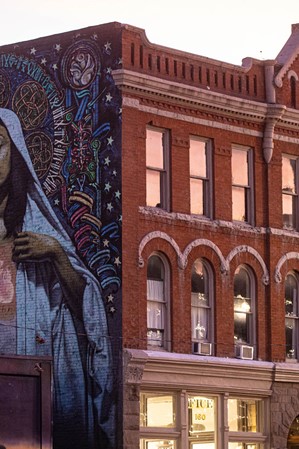A meticulously crafted building dominates the scene. The first floor showcases a façade of light-colored gray stone, featuring a sleek, rotating door composed of multiple panels that grant access into the building. Ascending above, two additional floors come into view. The second floor is constructed from a rich brown stone, seamlessly contrasted with gray stone trim. It flaunts a prominent, arched window with a rounded top, adding architectural character. The uppermost visible floor sports square windows symmetrically placed.

Adjacent to the edifice is a striking piece of mural art, although only partially visible. This artwork depicts a woman with long, dark hair and light skin, clothed in a flowing white robe. She stands before a backdrop resembling the night sky, filled with stars and vibrant hues of white, red, yellow, and green, giving the painting a mystical, spiritual aura. Unfortunately, the complete mural is cropped out, leaving the observer wanting more.

Hovering above the detailed structure is a dull, gray sky, thick with clouds, suggesting an overcast day.